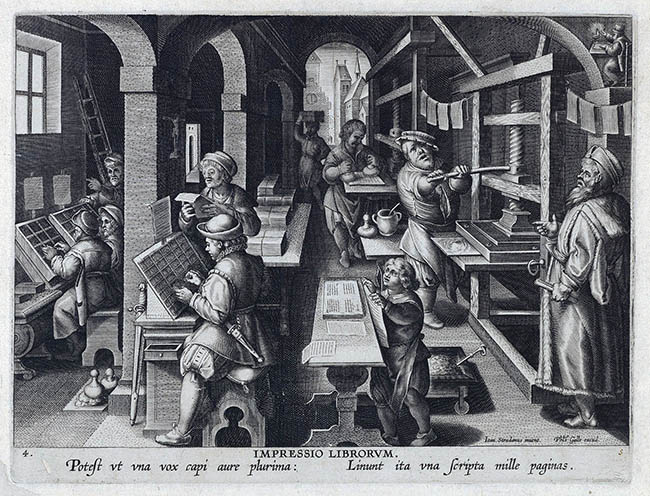This is a detailed black-and-white pen-and-ink drawing resembling a vintage postcard that illustrates a bustling scene inside an ancient print shop or scriptorium. The central focus is on numerous bearded men, all dressed in robes and hats typical of the 1400s to 1600s. They are engaged in various activities related to bookmaking and printing. One prominent figure operates a large screw press, seemingly pressing a plate, indicative of early printing techniques. Elsewhere in the room, individuals are seated at desks with slanted surfaces, possibly scribing or assembling documents. 

Another man holds a long stick, while yet another stands near an arched window, wearing a robe and hat. The room is adorned with hanging items, potentially drying print work, further emphasizing the artisanal nature of the scene. The background reveals more papers and a ladder, as well as a glimpse through a doorway to a town with tall buildings, adding depth to the illustration. Scatter on the floor are small objects resembling chess pieces, adding to the intricacy of the scene. The caption at the bottom reads "Impresso Libervorm," surrounded by Latin text, underscoring the historical and cultural context of the artwork. The image masterfully captures the essence of an old-fashioned workspace dedicated to the laborious task of bookmaking and printing.